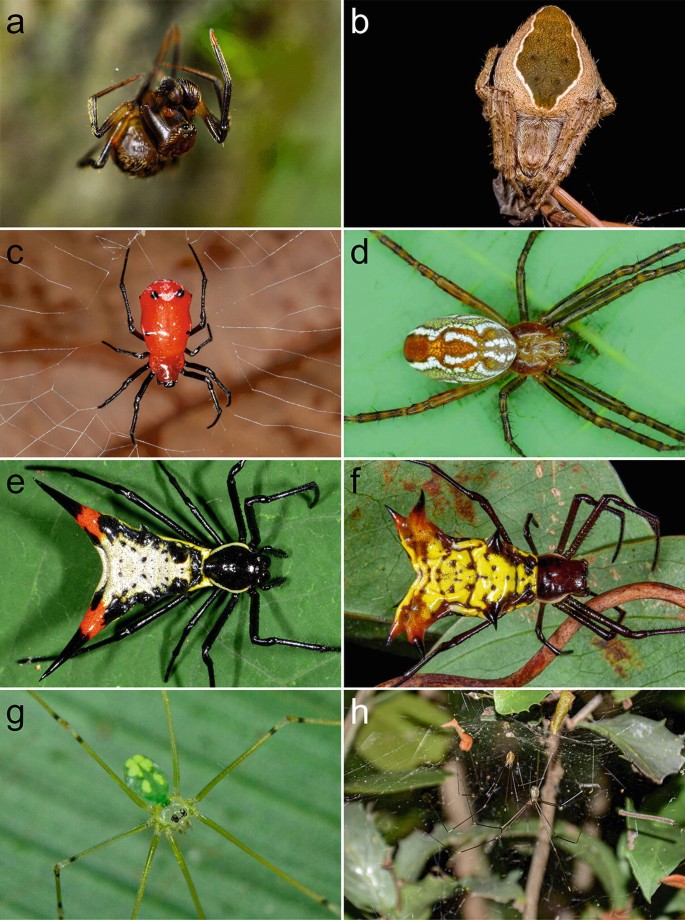The image showcases eight close-up photographs of spiders arranged in two columns and four rows, each labeled from A to H, starting from the top left to the bottom right. 

- **A**: A black spider with brown legs is set against a green blurry background, marked with a lowercase black 'a'.
- **B**: A brown spider with a darker brown back and tan sides, appears on a black background, marked with a lowercase white 'b'.
- **C**: A red spider with black legs, captured on a web, marked with a lowercase black 'c'.
- **D**: A brown spider with teal designs on its back, positioned on a green leaf, marked with a lowercase black 'd'.
- **E**: A peculiar black spider outlined in yellow, featuring a triangular, wing-like abdomen. It has a black shiny torso and legs, and is placed on a green leaf, marked with a lowercase black 'e'.
- **F**: A black spider with distinct yellow markings on its wide abdomen, on a green leaf, marked with a lowercase black 'f'.
- **G**: A green spider with light greenish-yellow dots on its back, appearing very long-legged, marked with a lowercase black 'g'.
- **H**: A gray, daddy long-legs type spider with a small body and long spindly legs, set against a backdrop of trees and branches with webbing, marked with a lowercase white 'h'.